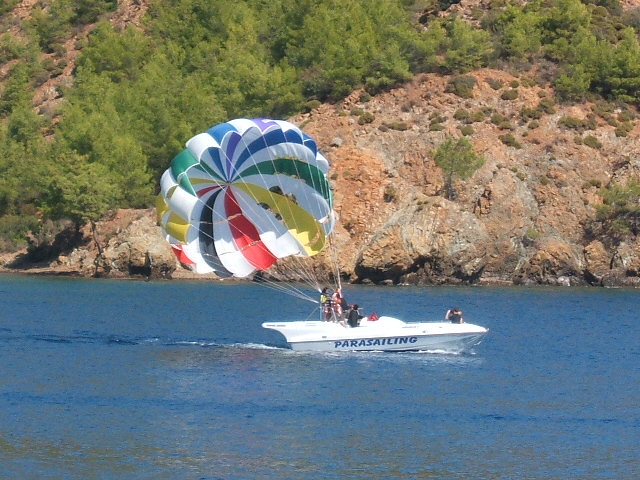This is an outdoor photograph capturing a vibrant parasailing activity on a tranquil blue lake. A small boat, prominently displaying the word "parasailing" on its side, moves from left to right across the calm water, creating gentle ripples. The boat is occupied by several people; one person sits at the front holding a camera, looking back at another who stands on the deck, ready to take off, attached to a gigantic, multi-colored parachute. The parachute, striped in white, green, blue, purple, yellow, and red, inflates behind the boat, preparing to lift its passengers. In the background, a majestic rock cliff rises high, crowned with a line of evergreen trees, adding a touch of rugged natural beauty to the scene.